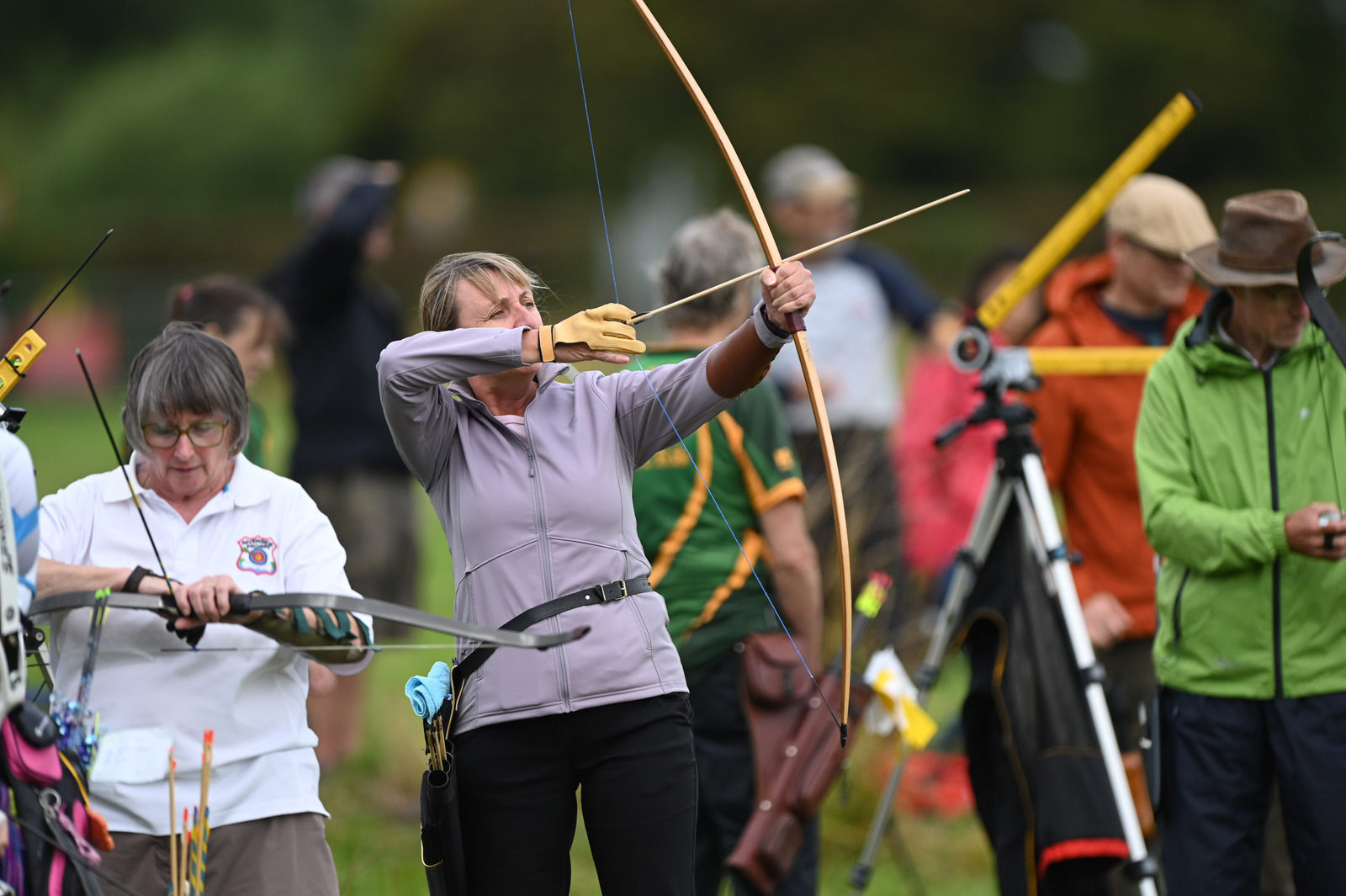The image is a well-lit, clear, color landscape photograph depicting an archery gathering. The central figure of the scene is an older woman, approximately 55 years old, with gray hair. She is prominently situated slightly below the center, facing the viewer while looking towards the upper right. Dressed in a purple jacket (or gray zip-front hoodie), beige/gold gloves, and black pants, she holds a bow, pulling back the string with an arrow (or white stick) positioned against it, ready to shoot. A black belt is visible across her waist.

To her left, in the bottom left corner of the photograph, is another woman in her 50s wearing a white polo shirt with beige trousers and dark-rimmed glasses. She is holding a black bow horizontally across her chest and focusing downward, stringing the bow with an arrow pointing toward the top left. She has a black protective wrist brace on her arm.

On the right side of the image, a man in a green jacket and a hat stands slightly out of focus. Additionally, a silver tripod is visible on the right side. The background becomes blurry and dark, emphasizing the clarity and well-lit nature of the main subjects. The photograph falls under the style of photographic representational realism, capturing the detailed and dynamic moment of the archery activity.